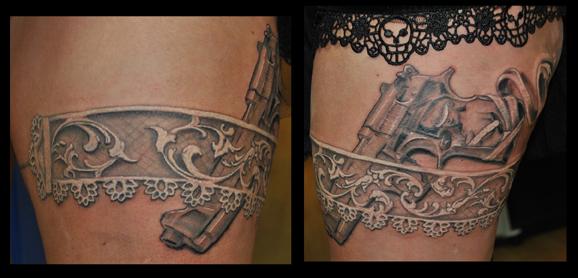This detailed photograph showcases two side-by-side images of an intricate tattoo wrapped around someone's upper thigh. The left image displays a delicate white lace garter belt tattoo encircling the leg, with a handgun tattooed as if tucked into the garter. Floral patterns are subtly incorporated into the lace design. The right image continues the visual story, illustrating how the tattoo completely encircles the thigh, revealing more black lace at the very top. The handgun is again visible, appearing to be holstered within the garter, with a ribbon tattoo wrapped around its base. The two images are separated by a black border, which also frames the entire composition, emphasizing the continuity and detailed artistry of the tattoo.